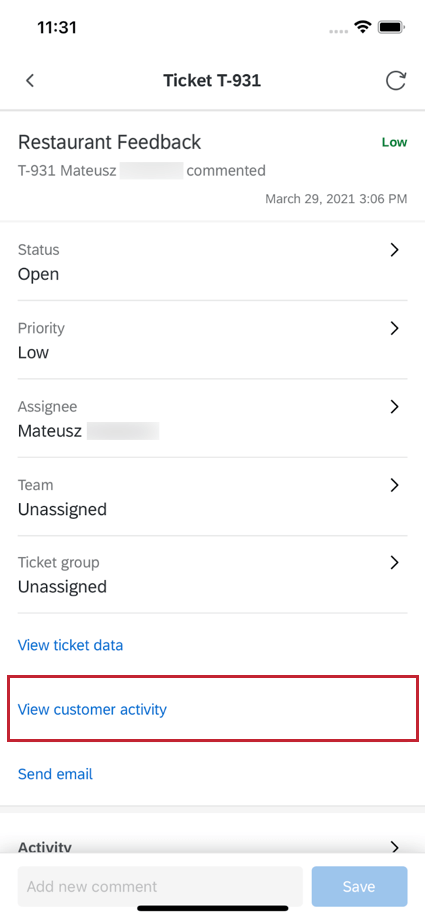The image depicted is a vertically rectangular screenshot of a mobile phone interface against a white background. At the top left corner, the black text shows the current time as 11:31. Adjacent to it on the right, icons display the Wi-Fi signal and battery level. Centered beneath this information is a notification reading "Ticket T-931," with a back arrow positioned to the left and a refresh icon to the right.

Following this header, the screenshot shows details of a ticket with a left-aligned indent, specifying that it is a restaurant feedback case labeled "T-931." The feedback is from an individual named Mateusz, written as "M-A-T-E-U-S-Z," who commented on the issue. Part of the comment is redacted. The timestamp indicates that the comment was made on March 29, 2021, at 3:06 p.m.

The interface presents a vertical list of ticket details, each accompanied by a forward arrow for further navigation. The list reads as follows:
- Status: Open
- Priority: Low
- Assignee: MATEUSZ, with the remaining part of the name grayed out
- Team: Unassigned
- Ticket Group: Unassigned

Below these details, there are blue hyperlinks offering further actions:
- View Ticket Data
- View Customer Activity, which is highlighted within a red, horizontally rectangular box
- Send Email

This detailed view provides a comprehensive snapshot of the ticket management system used, highlighting pertinent information and available actions for case resolution.